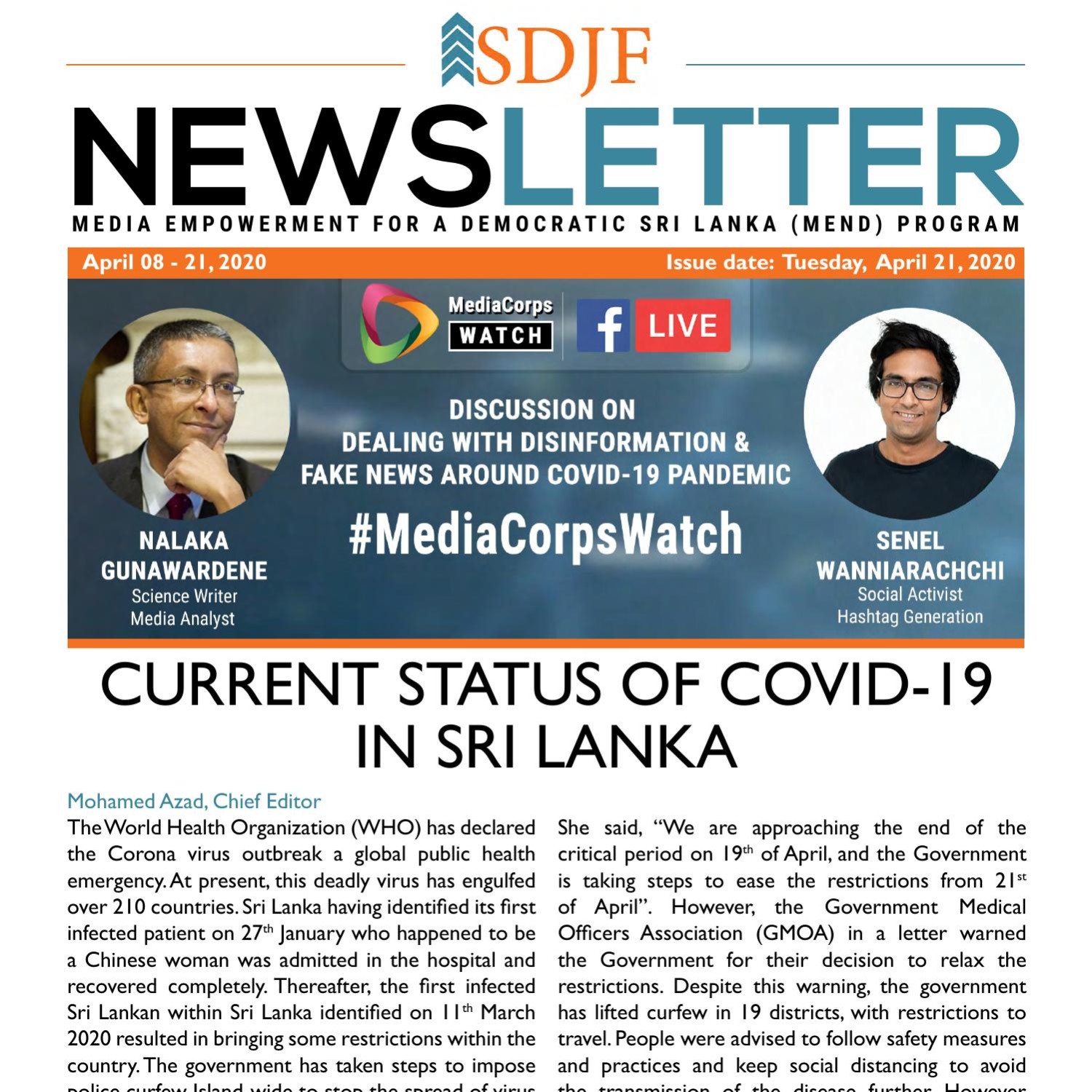The top left of the image features an orange bar with blue arrow lines pointing upwards. Black text reads "News" while blue letters spell out "Media." The black text also says, "Media Empowerment for a Democratic Sri Lanka (MEND) Program." The orange bar indicates the date range as "April 08-21, 2020," and notes "Issued Date: Tuesday, April 21st, 2020."

A ring of triangles in red, yellow, and green surrounds the centerpiece, promoting "MediaCord Watch" on Facebook Live. The discussion focuses on dealing with disinformation and fake news surrounding the COVID-19 pandemic. 

Panelists include:
1. **Nalaka Gunawardene** - Science writer and media analyst, shown with short hair, glasses, and holding his chin, wearing a tie.
2. **Vanir Nachchi** - Wearing glasses, short hair, and a black shirt.

The caption details the current status of COVID-19 in Sri Lanka:
- The World Health Organization has declared the coronavirus outbreak a global public health emergency.
- The virus has affected over 210 countries.
- Sri Lanka identified its first infected patient, a Chinese woman, in January, who was admitted to the hospital and recovered completely.
- The first infected Sri Lankan within the country was identified in March 2020.
- The government imposed restrictions to control the spread and announced easing of restrictions as of April 19th, lasting until April 20, 2020.